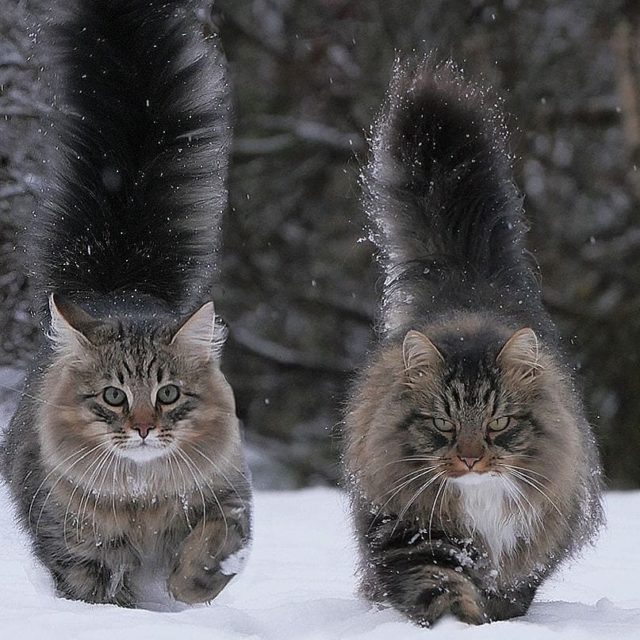This rectangular image, slightly taller than it is wide, captures two long-haired cats walking through a snowy outdoor scene towards the camera. These cats appear to be siblings, perhaps even Maine Coons, and have incredibly fluffy, puffed-out tails held straight up behind them. Their fur is a blend of brown and black markings, with distinguishing white chins. The cat on the left side, with green eyes and a heavier body, also features a white mouth and downward-slope whiskers. In contrast, the cat on the right has yellowish eyes, a white bib on its chest, and a face dominated by more black fur between the ears and wiry, sprawling whiskers. The background is blurred, revealing indistinct branches and brownish twigs, enhancing the focus on the cats who tread carefully through the snow, which reaches up to their shoulders. Their intense concentration on walking through the deep snow adds a touch of determination to the scene. The blurred black and gray background somewhat merges with their bushy tails, giving the impression of miniature lynxes navigating a winter wonderland.